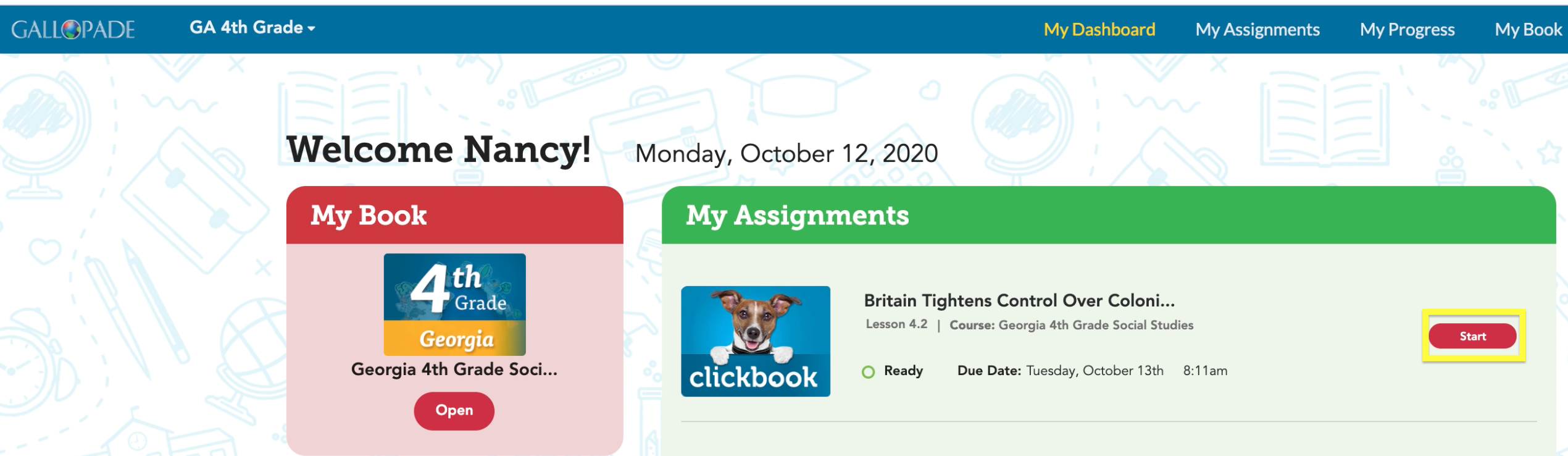This screen capture appears to be from an educational website designed for fourth-grade students. At the top of the page, there is a thin blue bar with the name "Galpain" in white font next to a circular, multi-colored logo. The bar also indicates "GA Fourth Grade" in white text, followed by an arrow pointing to the right. On the right-hand side of this blue bar, in yellow font, it says "My Dashboard," followed by three categories in white font: "My Assignments," "My Progress," and "My Book."

The main section of the website features a thin white strip with a series of hand-drawn style images including a globe with a landmass, a heart, a pen, a pencil, an alarm clock, a satchel or briefcase, an open book, and a graduation cap. 

Below the hand-drawn images, there are two mini windows. Above these windows, in black font, it reads "Welcome Nancy, Monday, October 12th, 2020." 

On the left window, with a dark red header strip that has "My Book" in white font, there is a pale pinkish-red background. This section includes a blue-and-gold square labeled "Fourth Grade Georgia," followed by "Georgia Fourth Grade S-O-C-I," although the text is cut off. Beneath this, there is a red box with the word "Open" in white font.

The right window has a dark green header strip that says "My Assignments" in white font, set against a pale green background. This section includes a blue square with the text "Click Book" and an image of a tan and white dog with a black nose. Below this description, the text reads "Britain Titans Control Over Colonial," which is also cut off. It mentions "Lesson 4.2 Course Georgia Fourth Grade Social Studies" and has a green circle with the word "Ready," indicating the assignment's due date is Tuesday, October 13th at 8:11 a.m. A red "Start" button with a yellow outline is located at the bottom of this section.